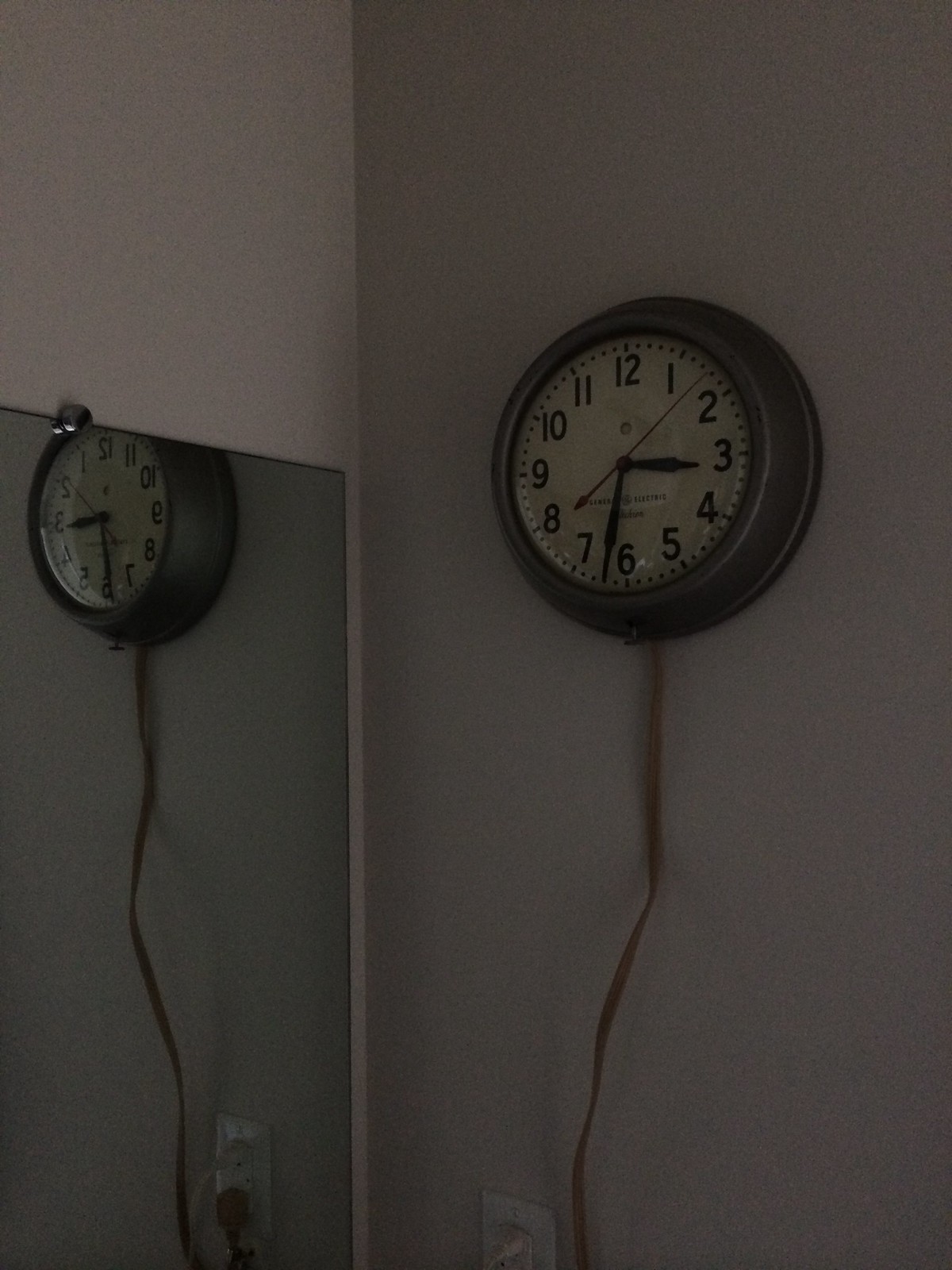This image captures a vintage wall clock mounted on a light-colored wall, located in the corner of a room. The clock, encased in a deep, brown housing with a large, round border reminiscent of a porthole, features a white face that has slightly yellowed with age. Black numerals and ticks mark the hours and minutes, while black hour, minute, and second hands indicate the time. 

Opposite the clock, a lower-hung mirror partially reflects the clock's image. Due to its positioning, the top of the clock is not visible in the mirror. The clock is powered by a brown cord, which is plugged into a white electrical outlet visible in the reflection within the mirror. This outlet also accommodates another white plug, highlighting the room's utilitarian detail.